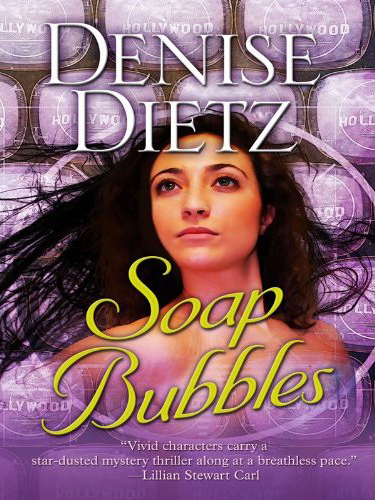This rectangular book cover illustration for "Soap Bubbles" by Denise Dietz features a central portrait of an enigmatic woman with long dark hair, dark brown eyes, thick black eyebrows, and pink lipstick, dressed in a pinkish-purple gown that cascades off her shoulders. Her pose conveys a sense of deep contemplation as she gazes upwards and away. The background consists of multiple rows of cylindrical purple shapes, each encasing the word "HOLLYWOOD" in faded white print, lending a repeating, stardusted pattern to the backdrop. At the top of the cover, the author's name, DENISE DIETZ, stands out boldly in white letters. Below the woman's portrait, the title "SOAP BUBBLES" is prominently displayed in vibrant yellow. Further down, a tagline in white reads: "Vivid characters carry a stardusted mystery thriller along at a breathless pace," a quote attributed to Lillian Stewart Carl. This captivating cover encapsulates the essence of a Hollywood-inspired, mysterious love story.